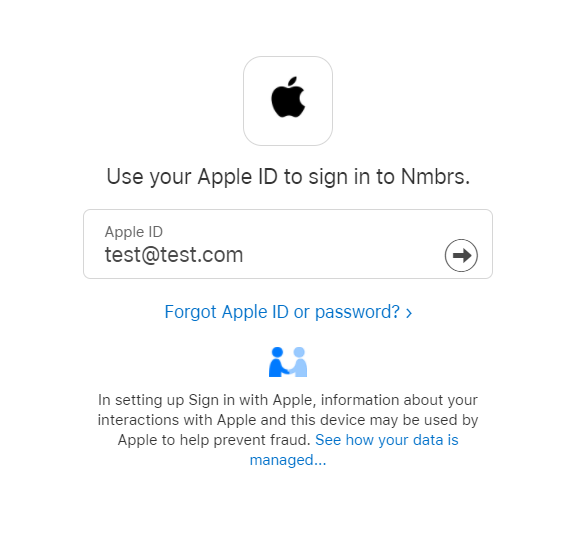In the image, a user is attempting to log into their Apple ID account. The login interface is characterized by a clean white background with a minimalistic design. At the top, a black Apple logo is prominently displayed against a white box. Below that, the interface prompts, "Use your Apple ID to sign into NMBRS."

The input field for the Apple ID is pre-filled with the placeholder text "test@test.com" in a light gray color, indicating where the user should enter their Apple ID. To the right of this input field, there is a right arrow button for signing in. Beneath the input field, a blue hyperlink reads, "Forgot Apple ID or password?", allowing users to retrieve their login credentials if needed.

Further down, there is an illustration of two people shaking hands; one figure is depicted in a darker blue while the other is in a lighter blue. Below this illustration, a black text message reads, "Instead of signing in with Apple, information about your interaction with Apple and this device may be used for Apple to help prevent fraud." This is followed by a blue link that says, "See how your data is managed..."

The interface is framed by a faint, light gray border that forms a square around the entire login section, maintaining the clean and organized look of the interface. Aside from the elements highlighted in blue and the black Apple logo, the rest of the login interface is predominantly white.